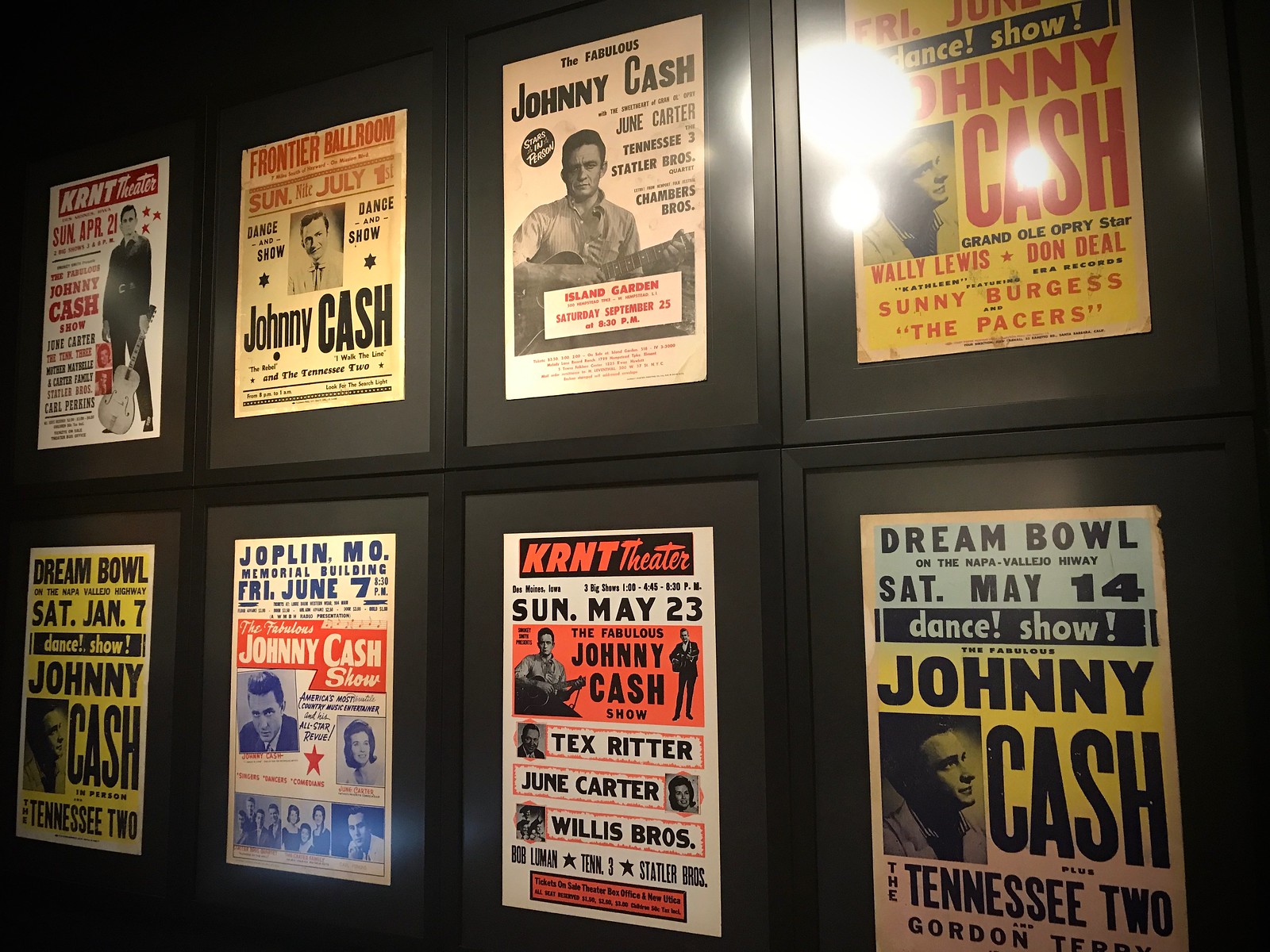This digital photograph captures a series of eight framed Johnny Cash posters, showcased against a black background that pays homage to the iconic "Man in Black." Each poster is a promotional advertisement for Johnny Cash's concerts, predominantly held at various venues in Tennessee and Missouri. The posters collectively feature vivid hues of red, white, black, yellow, orange, blue, and light blue. The posters display repeated texts of "Johnny Cash," and some include specific details, such as the leftmost poster for the KRNT Theater, where Cash is depicted holding a guitar. Adjacent to it is a promotional item for the Frontier Ballroom. The frames appear to be glass-encased, adding a reflective quality that blends with the ambient light, likely from three spotlights centered on the collection. At the bottom left, part of the photograph is illuminated by a reflected screen, possibly from a computer or television, adding a modern touch to the nostalgic display.